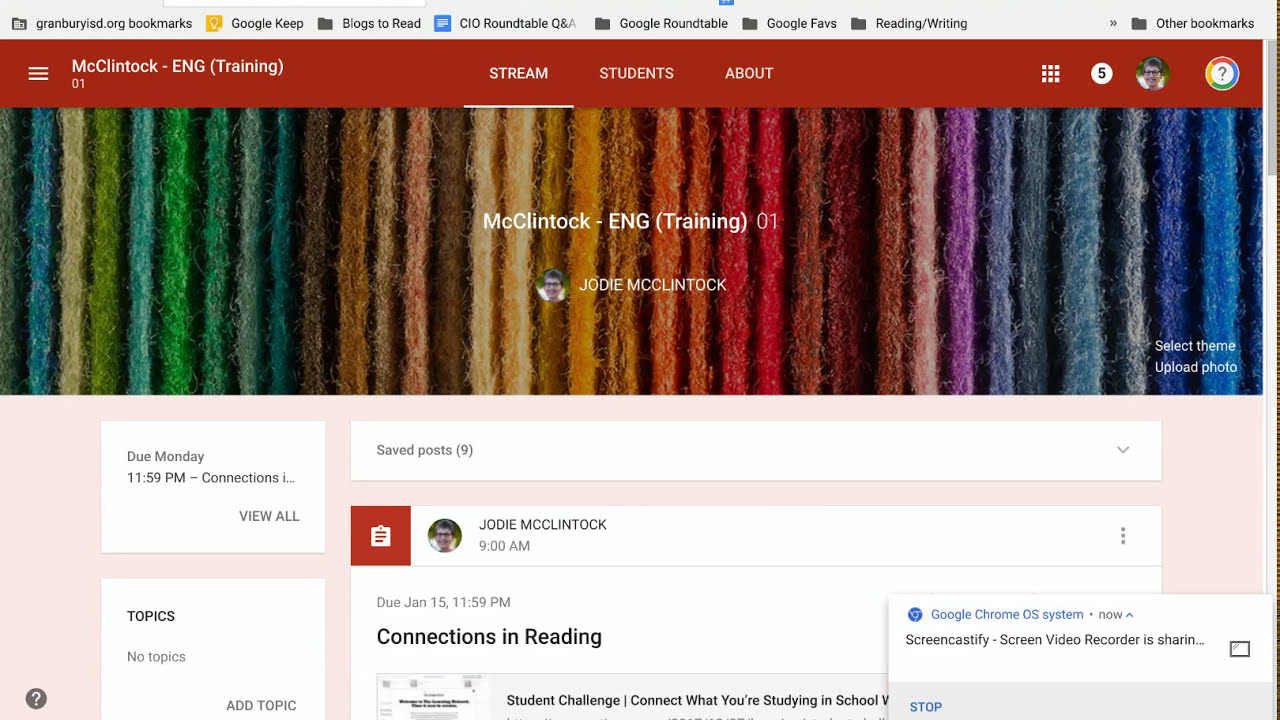The image is a screenshot of a web application displayed on a desktop or laptop computer monitor. The interface includes a bookmark toolbar along the top, with links such as Google Keep, Blogs to Read, Google Roundtable, CIO Roundtable, Google Faves, Reading, and Writing. Below the toolbar is the main interface of the web app, which features a red menu bar at the top, offering navigation links like Stream, Students, and About. The central part of the screen displays a large, hero-style image with the text "McClintock-ENGTRAIN," and immediately below this text, the name "Jody McClintock" appears along with a profile picture to the left. The background of the main section is a colorful, rainbow-like pattern with shades of red, purple, green, yellow, blue, and orange. Additional details include mentions of an ongoing class or training titled "McClintlock ENG Training 01," with specific reference to tasks such as "connections and reading" and a due date on Monday. The bottom right corner indicates that a screen video sharing feature is active, and the right side of the interface features a scroll bar. Additionally, a message says "screenshot successfully shared," indicating screen-sharing functionality.